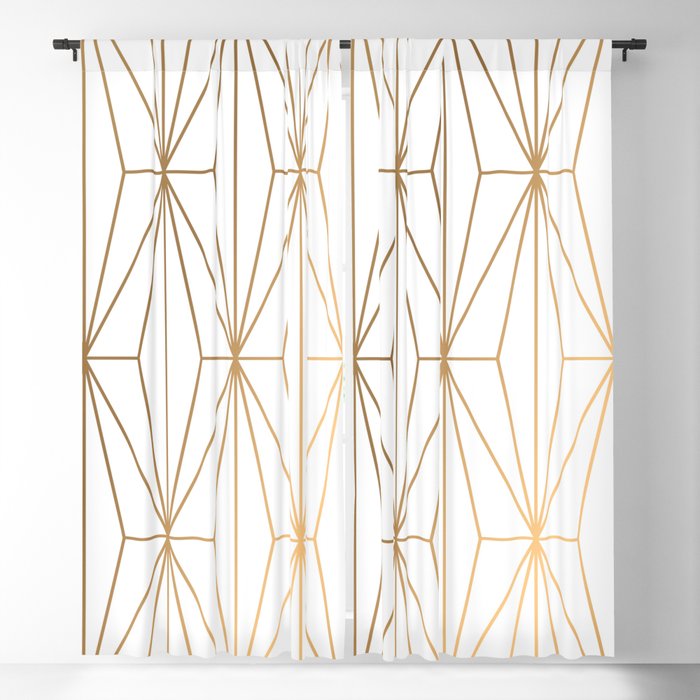The image depicts a vertical-rectangular photograph of curtains hanging inside a house against a wall that appears to be a shade of light gray. The curtains are mounted on a simple black metal curtain rod at the top. The curtains have a detailed design composed of diamond shapes created by intertwining lines; some of the lines are gold and form more continuous connections, while others are brown and sometimes disconnected. The background fabric of the curtains is white, and the repetitive pattern of diamonds spans the two separate curtain panels. The panels are hanging flat and possibly extend all the way to the floor, though the bottom part is not visible in the image. Light shines through the curtains, emphasizing their white background and intricate patterned design. The wall's color might also be influenced by lighting variations, giving off white, light gray, or possibly light blue hues.